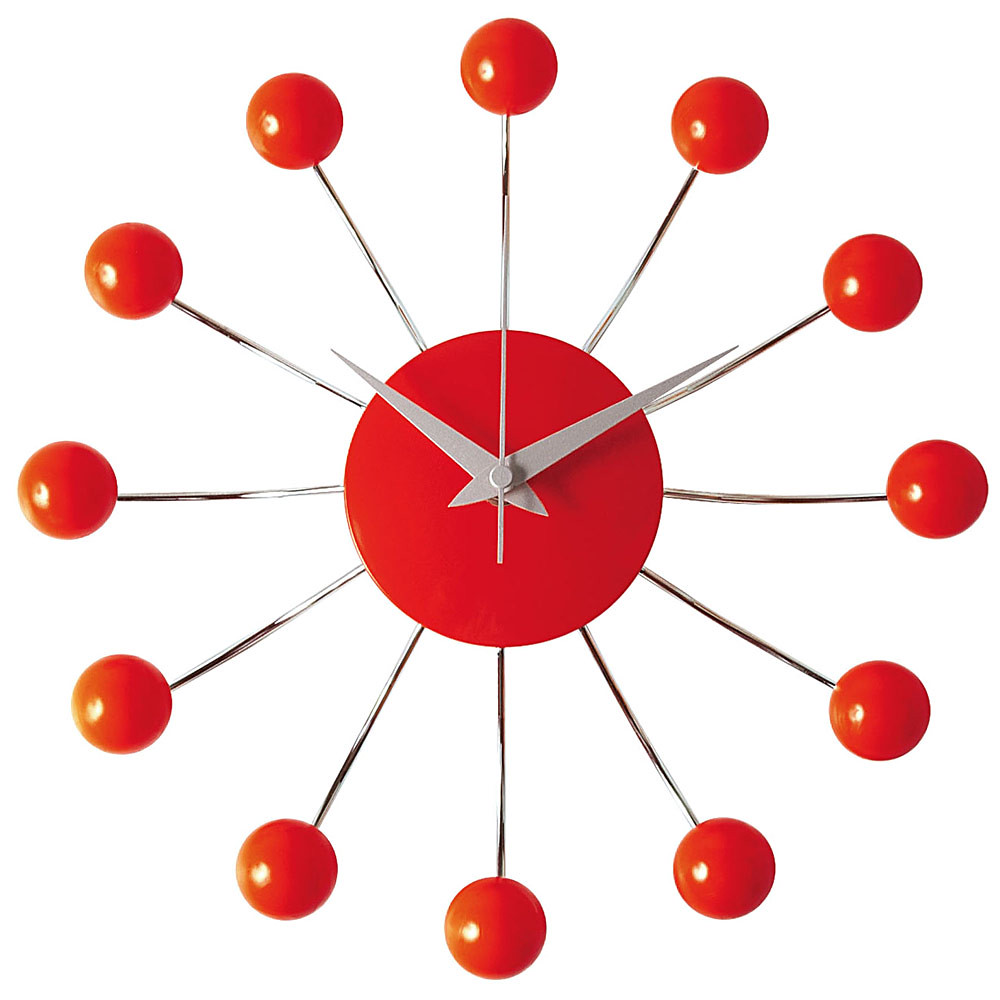This image showcases a unique and abstract clock design that teeters between the realms of photography and 3D modeling. The clock artfully adopts a sunburst motif, centered around a vivid, neutral red circle. From this nucleus extend sleek, silver metallic minute and hour hands, exuding a contemporary flair. Radiating outward, twelve slender metal spines replace traditional numerals, each tipped with a glossy, round red sphere. These spheres catch the viewer's eye, each adorned with a subtle reflection of artificial light highlighting their left side, hinting at a nearby lamp outside the frame. The intricate interplay of light and materials in the design suggests a masterful blend of artistic innovation and functional elegance.